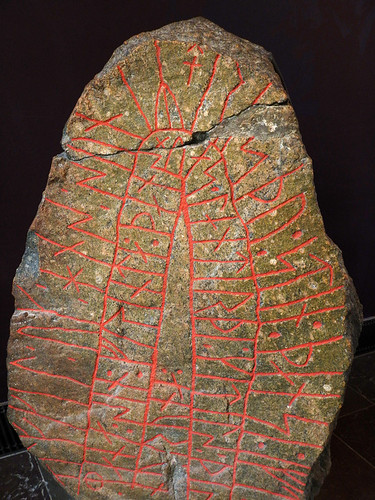In this striking image, we see an oval-shaped rock adorned with intricate carvings, standing upright against a very dark background. The rock exhibits a mix of yellow, brown, orange, and gray hues, along with some areas that appear slightly green, suggesting the presence of mold or weathering. Numerous red carvings span across the rock's surface, dominated by a central design resembling an umbrella or canopy. This central carving consists of lines that converge to form an outer layer and an inner layer, both red in color. Two columns of red rectangles rise up the middle of the rock and curve into each other at the top, reminiscent of crisscrossing ladders. Additional lines extend outward from these central columns toward the edges of the rock. Notably, the top of the rock appears to have been broken off and reattached, evidencing visible cracks. In the background, a hint of white branches or possibly scratches is visible on the left side, adding an enigmatic element to the composition.